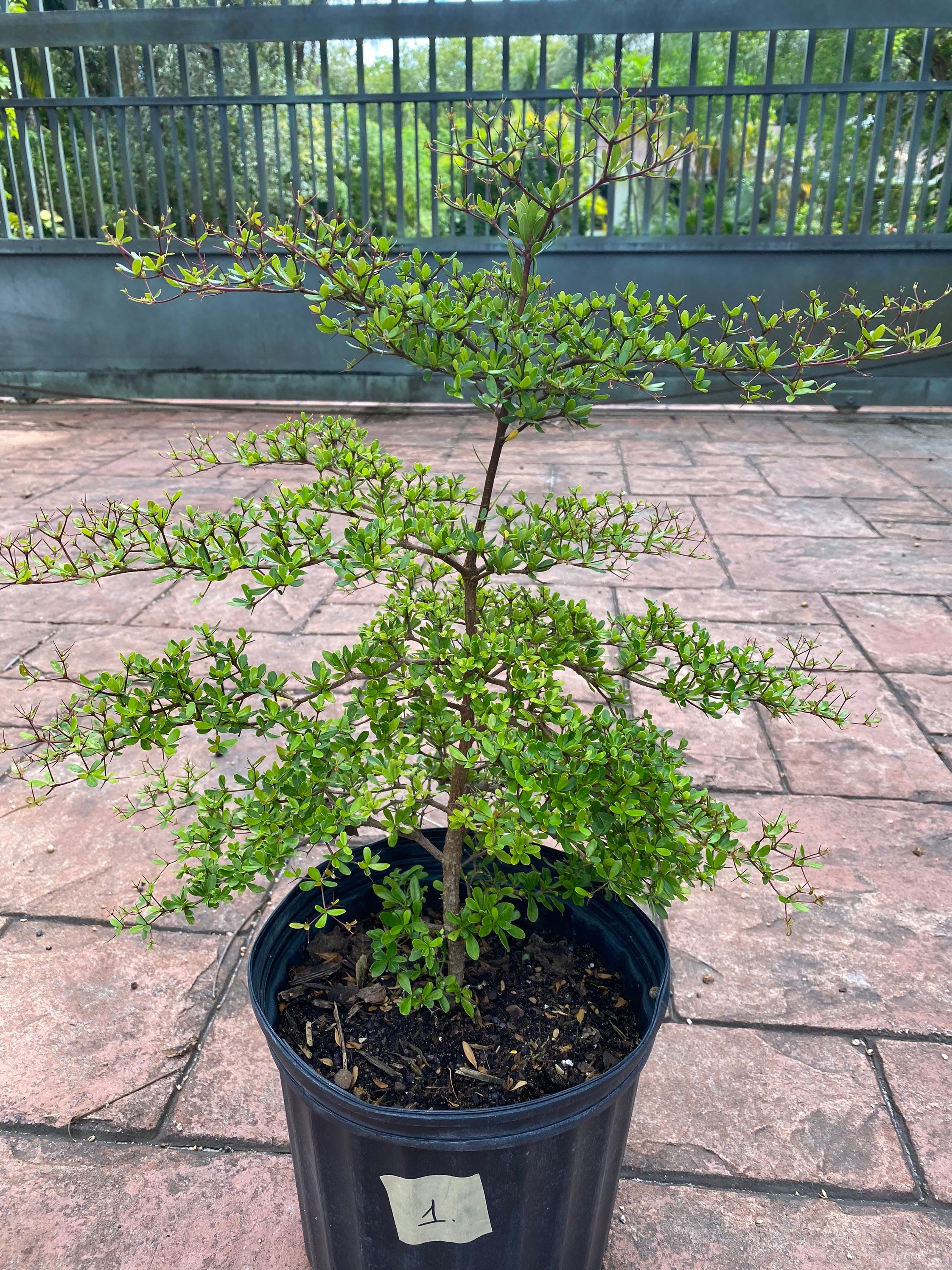This photograph, taken outdoors during daytime, captures a young plant still in its early growth stages, housed in a black, almost plastic-like pot. The pot stands on a red brick sidewalk, with a piece of tape bearing the number "1" affixed to its side. The plant itself is a small tree or bush, characterized by a central twig-like stem with several branches holding a few tiny green leaves. Behind the pot, a dark green, almost steel-like iron gate encloses the area, with many trees visible beyond, suggesting a semi-enclosed environment, possibly featuring overhead cover due to the diffused sunlight.